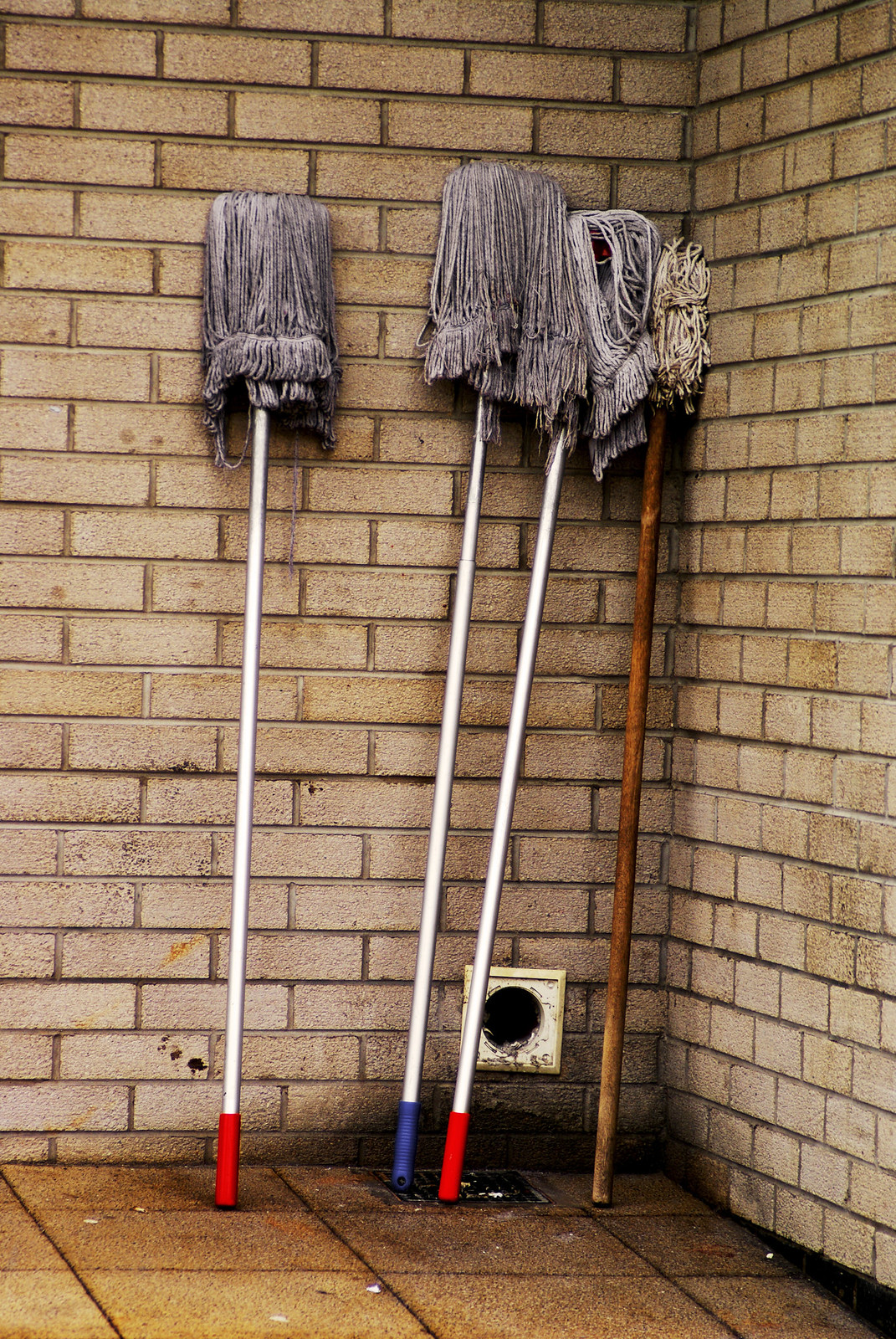In the photograph, four mops are leaning against the corner of a room with brick walls. The bricks, originally white, appear dirty with gray and yellowish stains. The mops include three with metallic silver handles and one with a dark brown wooden handle. The silver-handled mops have grips colored red, blue, and red from left to right, respectively. Their ragged, dark gray heads hang down, contrasting with the slightly shorter, whitish string mop head on the wooden-handled mop. The floor beneath the mops is tiled and shows signs of dirt and possible mold, with variations in black and brown hues. A circular drainage vent with a silver border is located near the corner, just under the middle two mops.